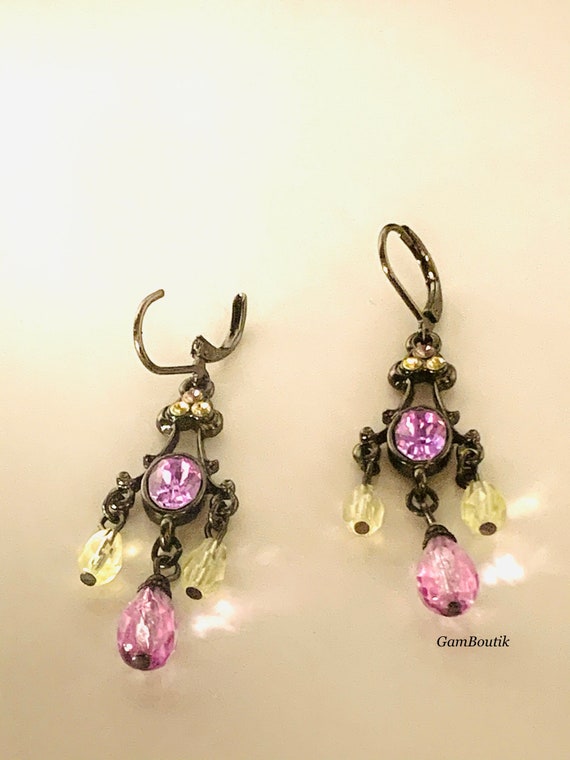This is a detailed photograph of an ornate pair of vintage-style earrings designed for non-pierced ears, showcasing their intricate craftsmanship. The earrings, made from a pewter-colored metal that looks like a dark antique gold, are adorned with an array of gemstones. Each earring features a large central pink gemstone, complemented by three white crystals near the top clasp. The base of the main gemstone is accented with multiple hanging crystals, consisting of two white crystals and two yellow crystals, arranged in a delicate trifecta pattern, adding to their chandelier-like appearance. 

The background of the image is a plain, neutral beige with light reflecting through the hanging crystals, casting subtle glimmers onto the surface. The left earring is depicted with its clasp open, while the right one shows the clasp closed. Below the right earring, in small text, is the label "GAM Boutique" (G-A-M B-O-U-T-I-K), indicating the creator of these stunning pieces. The composition of the photo highlights the earrings' reflective quality and intricate details, creating an overall effect of elegance and vintage charm.